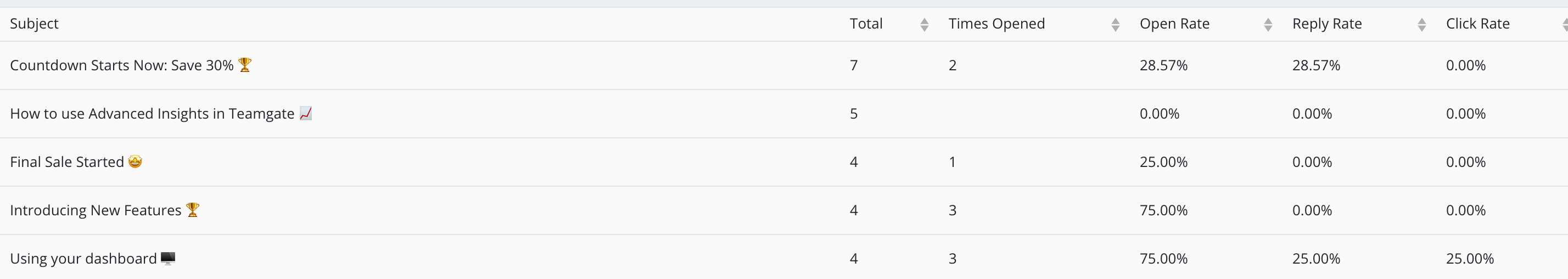The image displays a detailed chart on a gray background, showcasing various performance metrics for different email subjects. 

1. **"Countdown Starts Now - Save 30%"**
   - **Total Sends:** 7
   - **Times Opened:** 2
   - **Open Rate:** 28.57%
   - **Reply Rate:** 28.57%
   - **Click Rate:** 0.00%

2. **"How to Use Advanced Insights"** 
   - **Total Sends:** 5
   - **Times Opened:** (Blank)
   - **Open Rate:** 0.00%
   - **Reply Rate:** 0.00%
   - **Click Rate:** 0.00%
   - *Note:* The subject text is in smaller font and may include the word "TeamGate."

3. **"Final Sales Started"**
   - **Total Sends:** 4
   - **Times Opened:** 1
   - **Open Rate:** 25.00%
   - **Reply Rate:** 0.00%
   - **Click Rate:** 0.00%

4. **"Introducing New Features"**
   - **Total Sends:** 4
   - **Times Opened:** 3
   - **Open Rate:** (Information incomplete in provided details)

Each subject line in the chart is evaluated based on the total number of emails sent, how many times they were opened, their open rate (percentage of recipients who opened the email), reply rate, and click rate.